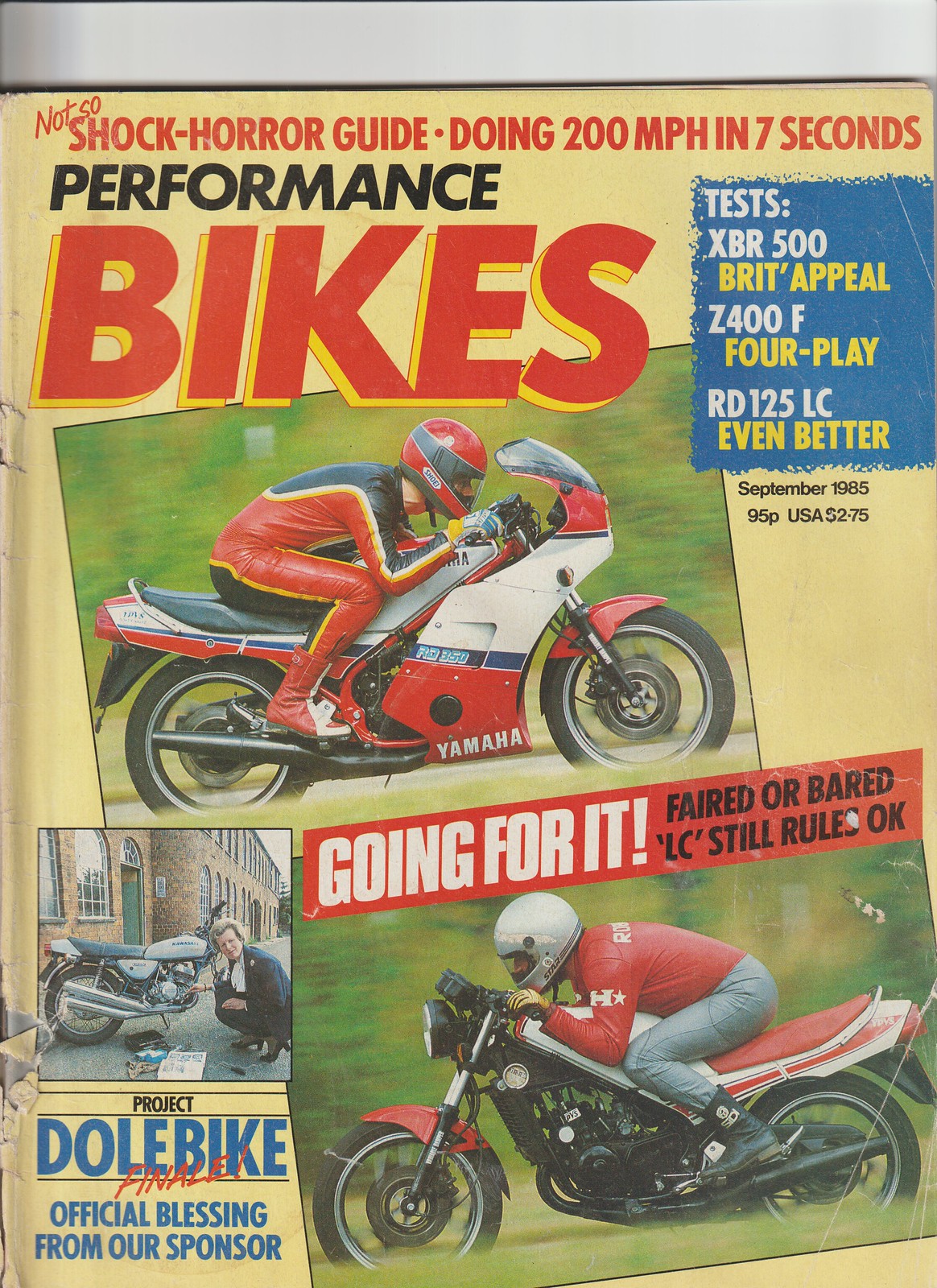This image is a cover of an old, vintage 1985 motorcycle magazine titled "Performance Bikes." It features a cream-colored background with striking red and black typography, predominantly employing bold and italic styles. The top of the cover reads "Not So Shock-Horror Guide: Doing 200 MPH in 7 Seconds" in dynamic red lettering, with "Not So" in italicized font. Below this headline, the word "Performance" is in bold black italic, and "Bikes" appears in bold red italic with a yellow drop shadow.

On the right side of the cover, there's a blue text box with white and yellow font detailing technical tests: "Tests: XBR 500" in white and "Brit Appeal Z 400 F" and "For Play RD 125 LC Even Better" in yellow. The lower section displays multiple images — two of bikers in action and one of a man kneeling beside a motorcycle with tools laid out in front. The prominent image features a rider in a red and black striped outfit, red helmet, and riding a red and white Yamaha bike.

The bottom section includes additional elements: on the bottom right, a heading that reads "Going For It" in bold white letters accompanies another biker in a silver helmet, red jersey, and silver pants on a red motorcycle. Next to this photo is the caption "Fared or Bared: LC Still Rules." The bottom left corner contains the text "Project Dole Bike" in all blue caps, followed by "Finale" in red with an exclamation point. This magazine cover, rich in colorful imagery and vivid typography, perfectly epitomizes the vibrant, high-adrenaline spirit of 1980s motorcycle culture.